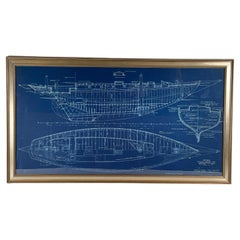The image is a detailed and intricate architectural drawing of the hull of a ship, depicted horizontally within a rectangular frame. The background is a vivid blue, characteristic of a blueprint, while the drawing itself is rendered meticulously in white, showcasing all lines, dimensions, and key structures of the vessel. The ship's design appears to display different views or parts of the hull, akin to an anatomical sketch highlighting its essential components. The frame surrounding the blueprint is predominantly gold with hints of silver, giving it an elegant, collector's item appearance. The overall composition suggests a profound focus on the technical and structural aspects of the ship's construction.